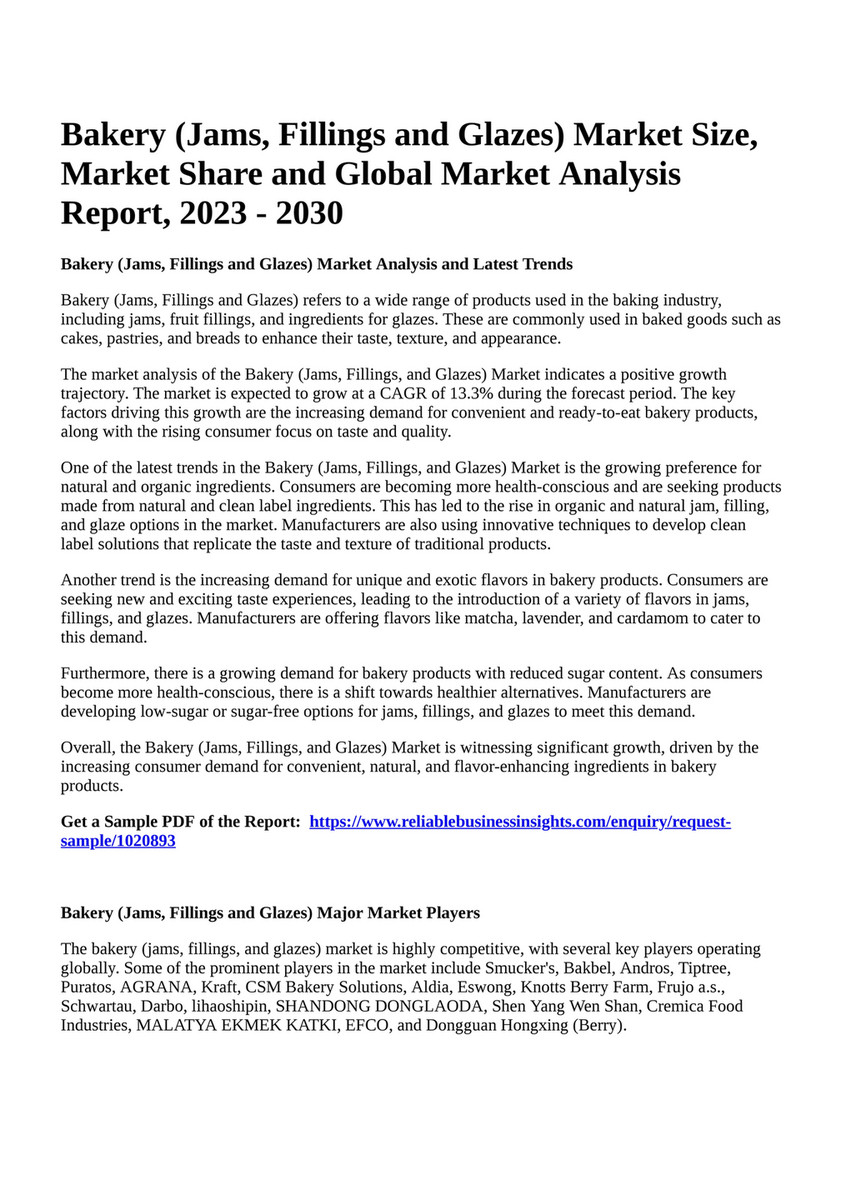The black and white image is a vertical promotional material displaying a detailed market research report. Titled "Bakery Jams, Fillings, and Glazes Market Size, Market Share, and Global Market Analysis Report 2023-2030," it presents an in-depth analysis of the market trends and growth trajectory for these bakery additives. The document includes six concise paragraphs, each delving into aspects such as market size, share, and latest trends. It highlights the increasing demand for convenient bakery products and a rising consumer focus on quality and taste, predicting a growth rate of 13.3% for the sector during the forecast period. At the bottom of the image, there is a link in blue inviting viewers to "Get a sample PDF of the report."